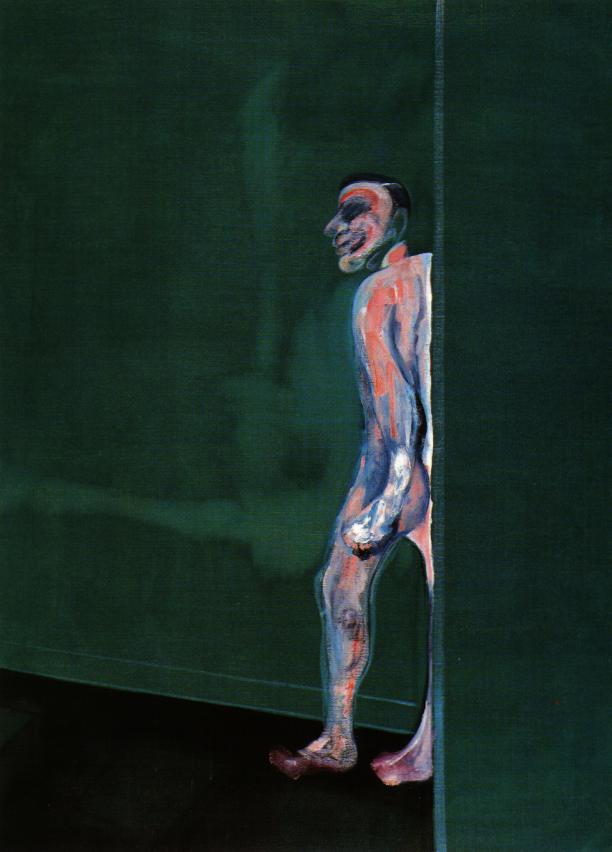The image appears to be a dark and unsettling oil painting set within a dimly lit room with dark forest green walls and a black floor. Dominating the scene is a disturbing figure, possibly a ghost or demon, with black hair and a frightening face, featuring a creepy smile and a large nose. The figure stands in a side profile with its left arm towards the viewer, menacingly emerging from a vertical line on the right third of the image. Its skin is a haunting marbled blend of blue, salmon pink, white, and purple, with visible muscles and an almost skeletal appearance on its hands. The lifeless eyes are black, and there is a striking dark salmon paint over one of them. This eerie figure stands out starkly against the shadowy, featureless backdrop, adding to the overall sense of dread and fear.